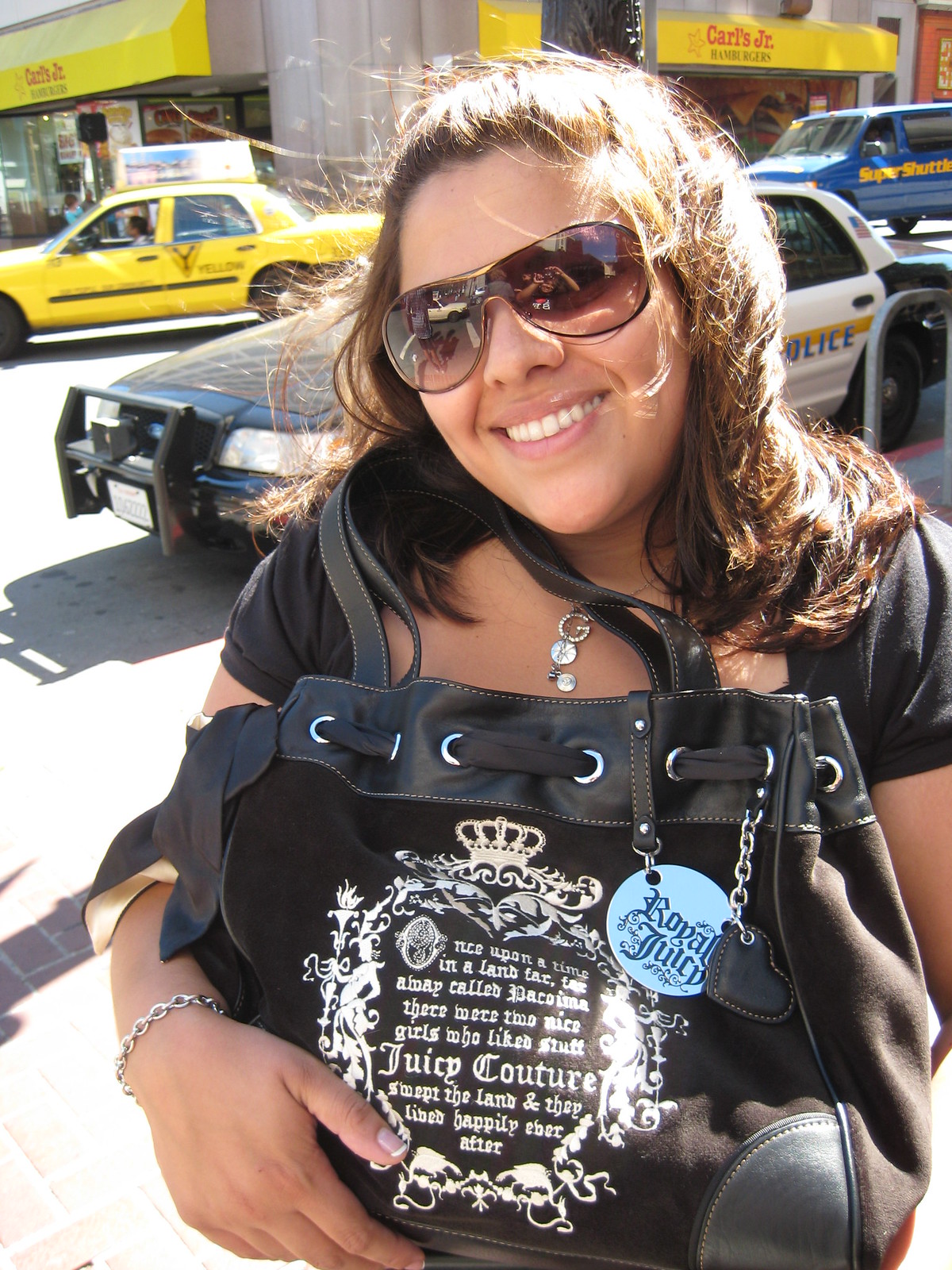In this vibrant city scene, a woman with shoulder-length brown hair, partially pinned up, stands confidently smiling at the camera, framed by the warm sunlight. She wears thick sunglasses and a black shirt, accentuated by a silver necklace featuring the letter "G." In her hands, she holds a stylish black Juicy Couture handbag adorned with intricate details, including white text that reads, "Once upon a time in a land far, far away called... nice girls who liked Juicy Couture and lived happily ever after," along with various keychains like a black heart and a blue circle. The bustling urban background reveals a mix of everyday life: a black-and-white police car is parked nearby, a bright yellow taxi cab drives past, and a blue van with "Super Shuttle" written in yellow speeds by. Adding to the city's character is a Carl's Jr. restaurant, easily identifiable by its yellow awning with red text and a hamburger logo crowned by a star. The blue sky and sunlit asphalt complete this lively daytime snapshot.